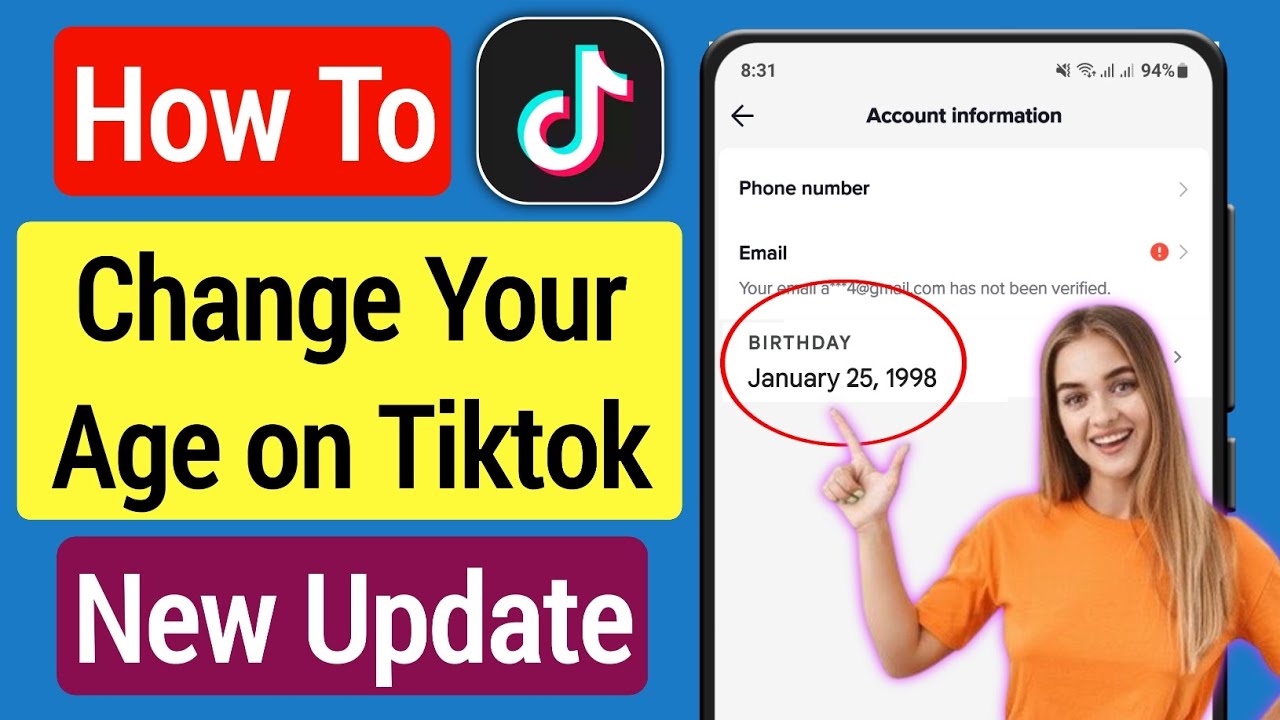This image is a detailed screenshot of a web page designed to guide users on how to change their age on TikTok, showcasing the new update. The web page features several distinct elements:
- A predominantly blue background.
- A red box with white text titled "How To."
- The TikTok logo beneath the red box.
- A yellow box with black text that reads "Change Your Age on TikTok."
- A burgundy box with white text stating "New Update."

To the right of these descriptions is an enlarged smartphone screen displaying a TikTok account settings page. The smartphone screen details include:
- A timestamp of 8:31.
- A sound icon, Wi-Fi icon, and a battery icon at 94%.
- A left-facing arrow labeled "Account Information."
- Below the arrow, text indicating "Phone Number" with a right-facing arrow next to it.
- An option labeled "Email" indicating "Your email email@gmail.com has been verified" with an attention symbol and right-facing arrow.
- Most notably, a red circle highlighting "Birthday January 25, 1998."
- A young woman, dressed in a yellow-orange T-shirt with brownish blonde hair, is pointing to the circled birthday information.

This comprehensive visual aide assists users in navigating the steps needed to update their age on TikTok, underscoring the most recent changes to the platform's settings interface.